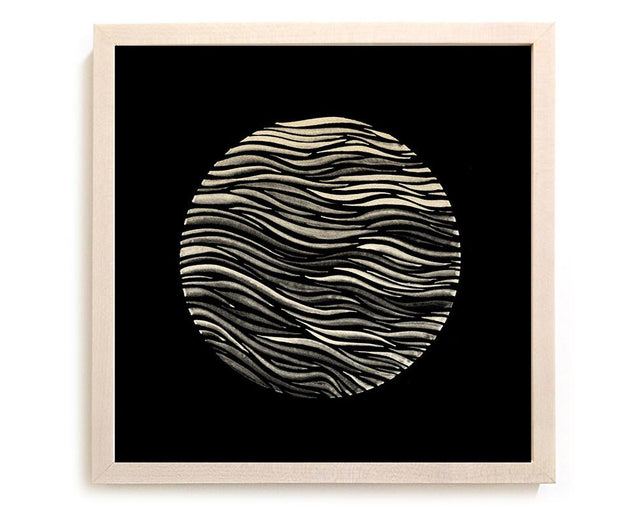The artwork features a striking black circle adorned with intricate beige, tan, and gray squiggly lines, creating an eye-catching and textured appearance. This central circular element, resembling either a stylized planet or an abstract globe, rests on a jet-black background, heightening the visual contrast and making the muted tones within the circle stand out. Adding a subtle yet impactful border is a very light pink, cream, or tan square frame that elegantly encapsulates the entire piece, enhancing its aesthetic appeal with a harmonious blend of colors. The combination of the detailed squiggly lines, the stark black background, and the delicate light-colored frame results in a visually compelling and unique piece of art that is both simple and profoundly pretty.